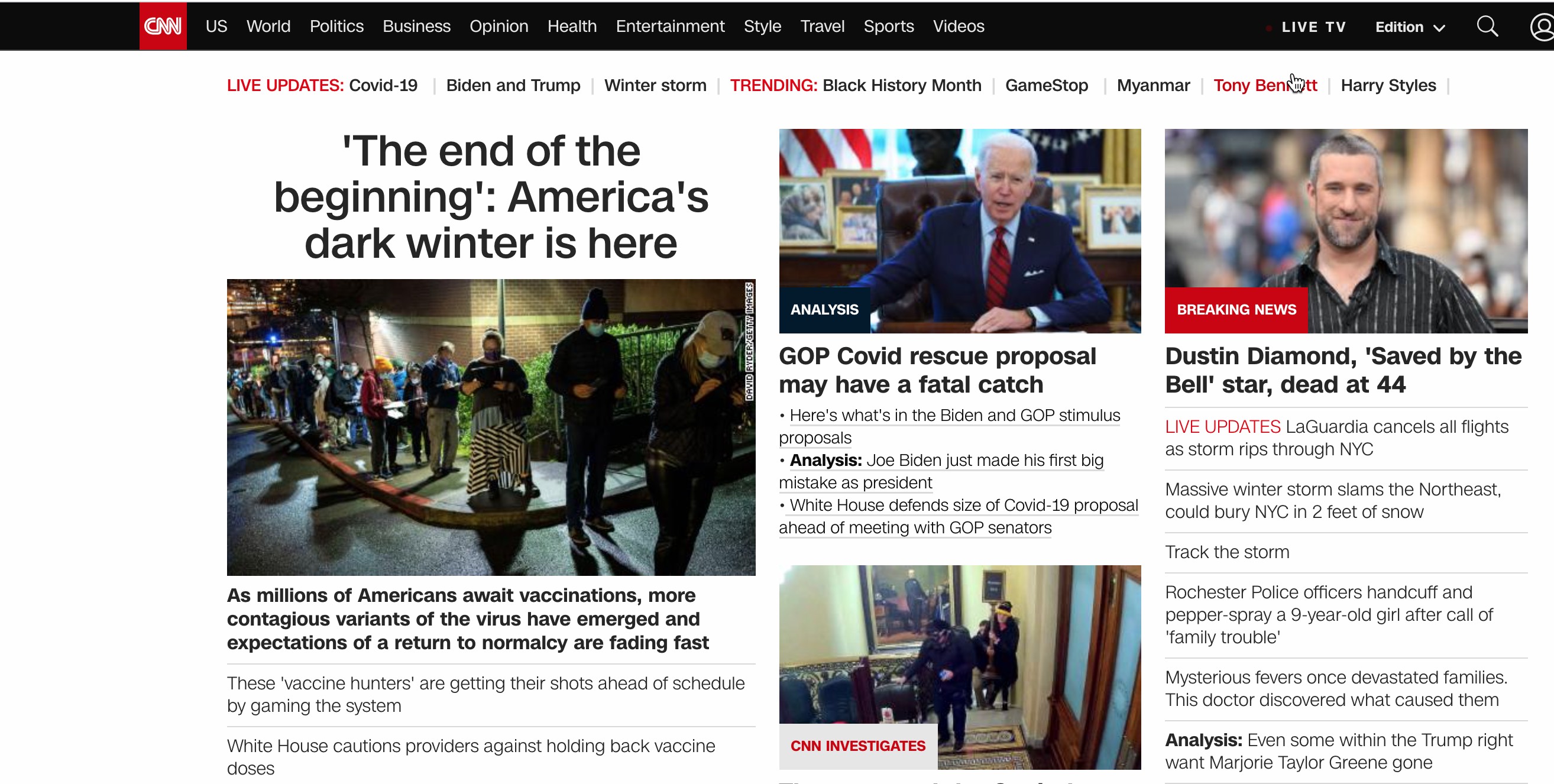The CNN website homepage features a striking contrast of colors with a prominent black top border and a white background for the main content area. Along the top black bar, there is a red tab with the white text "CNN" followed by white text menu items including U.S., World, Politics, Business, Opinions, Health, Entertainment, Style, Travel, Sports, and Videos. On the far right, icons for profile and search are visible, alongside menu options for Edition, Live TV, also in white.

Just below this header, in the white section, a horizontal red "Live Updates" tab followed by a series of trending topics including COVID-19, Biden-Trump, Winter Storm, Black History Month, GameStop, Myanmar, Tony Bennett, and Harry Styles, each separated by thin divider lines, dominate the top section.

Three major news articles are presented side by side. The first features a headline: "The End of the Beginning: America's Dark Winter is Here," accompanied by an image of people waiting outside in the dark. The second article shows Joe Biden in the Oval Office with the bolded title: "GOP COVID Rescue Proposal May Have a Fatal Catch." Below it, another photograph displays people in a hallway. The third section features an image of Dustin Diamond with a "Breaking News" tag in the upper left corner, followed by relevant information beneath.